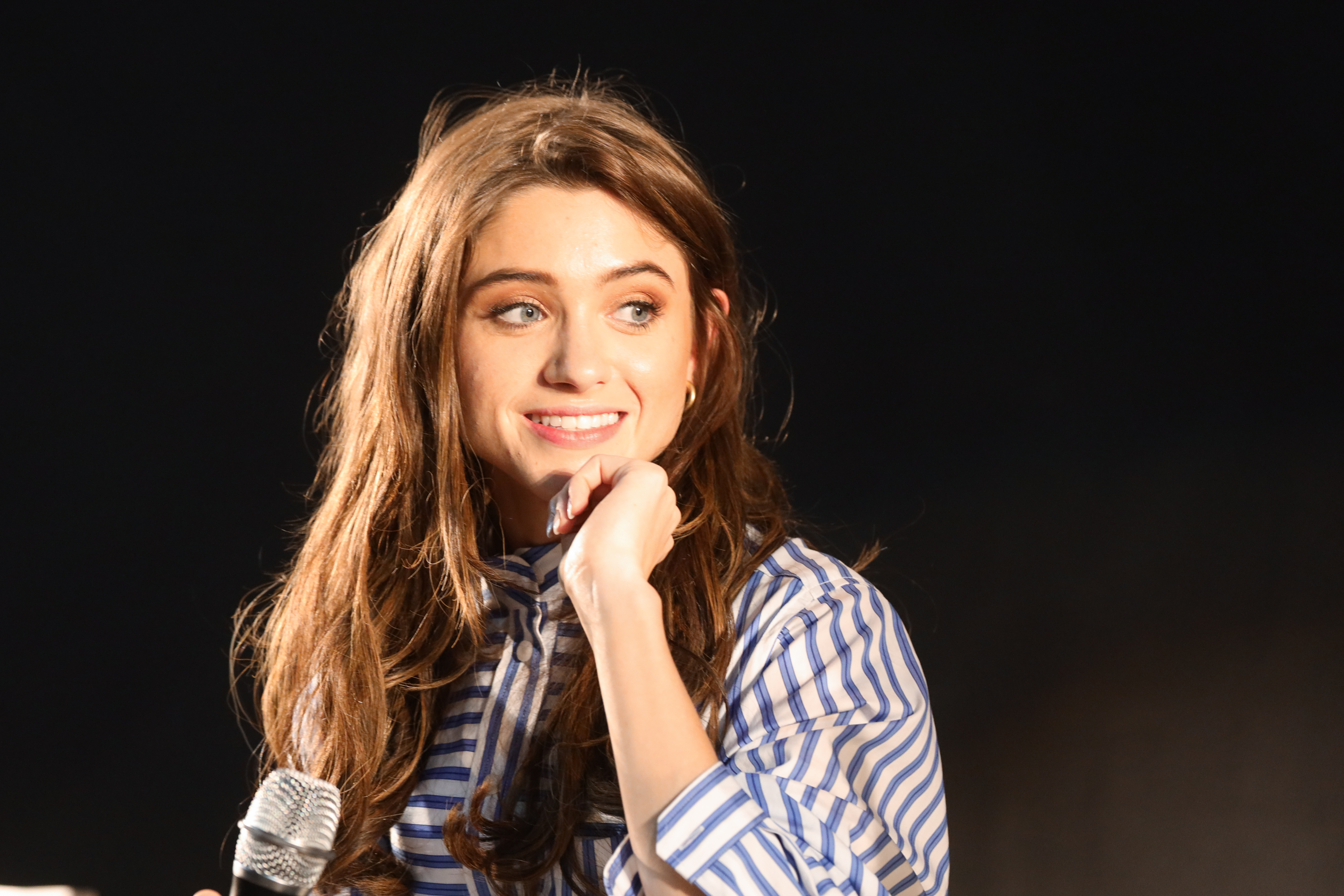In this image, a young woman is centrally positioned against a predominantly black backdrop, which appears to be an indoor setting possibly during a performance. The woman has a round face framed by long, wavy, and tousled brown hair that looks fluffy and messy. Her expressive blue eyes, enhanced by a touch of eye makeup, are looking off to the right. She is smiling warmly, revealing the top row of her teeth. The woman is dressed in a white shirt adorned with blue stripes. Her left arm is bent at the elbow, with her hand resting against her chin in a thoughtful yet cheerful pose. A silver microphone, seemingly held by her, extends from the bottom left of the image towards her. The background is diffused in darkness, with a strong light source from the left illuminating her face, highlighting her cheeks and forehead, and making her the focal point of the composition. There are no other visible objects or text in the photograph.